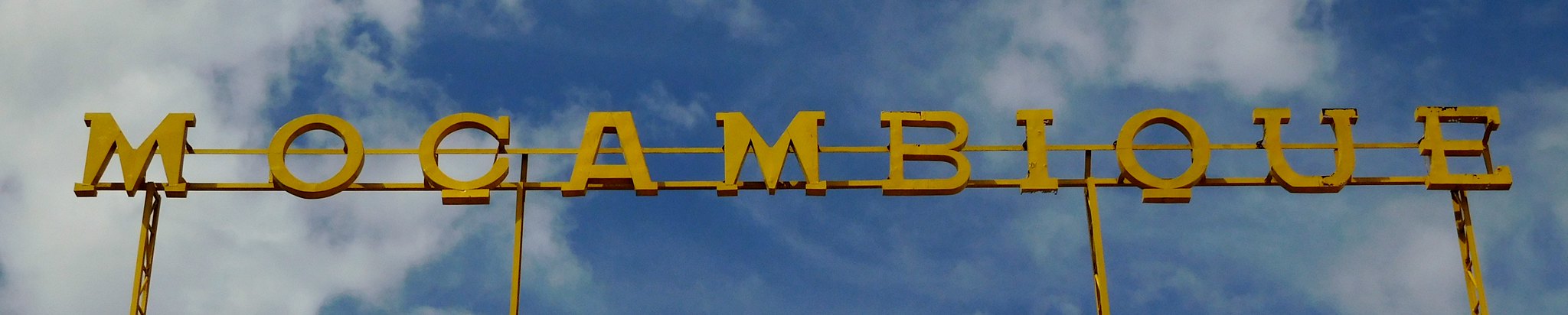This is a very large, rectangular sign that reads "Moke and Beak." It is painted in a vibrant yellow and supported by four poles. The letters, also yellow, are affixed to two horizontal metal beams. There’s a small dashed line symbol beneath the letter "C." The photograph is taken from a low angle looking up towards a clear blue sky dotted with puffy white clouds. The sign's metal structure shows signs of rusting, particularly evident on the right pole and the letters to the right. The overall composition highlights the sign against the bright sky, with its intricate details and weathered texture clearly visible.